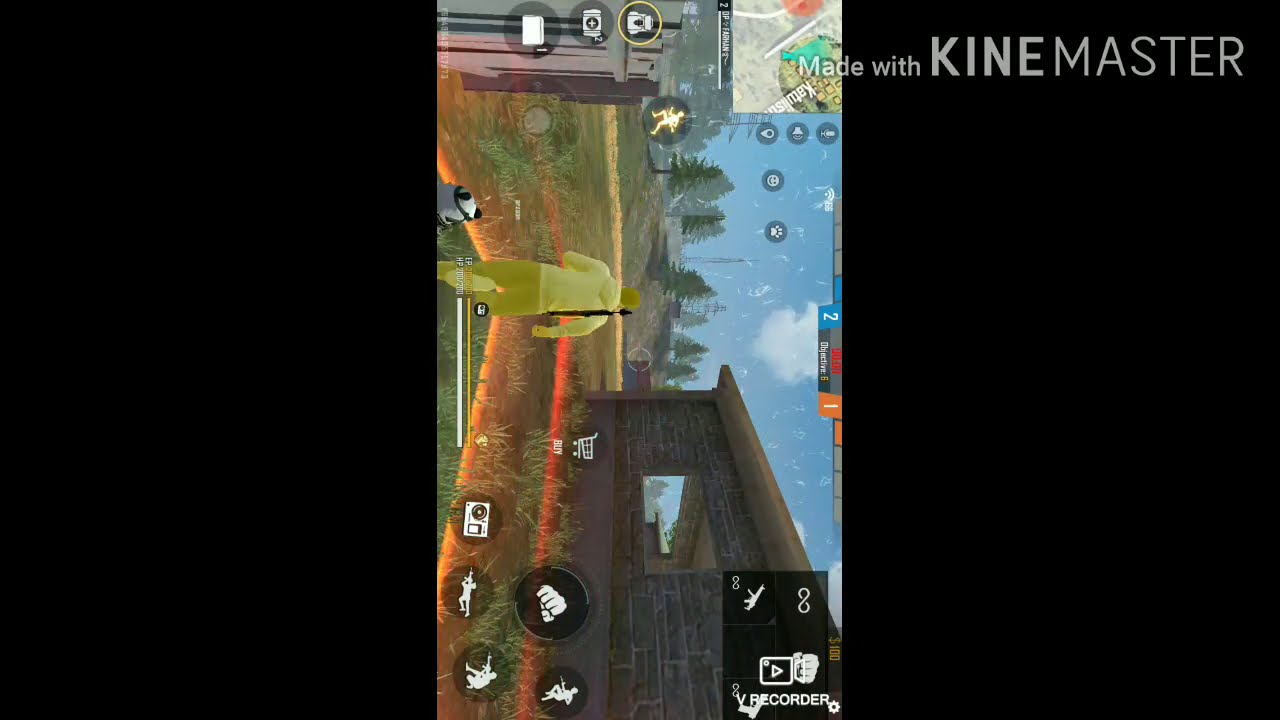The image showcases a digital scene reminiscent of a video game screenshot, rotated 90 degrees to the right. Centered in the frame is a main character, dressed in a gray hoodie and colored yellow, walking away from the viewer. To his right, there's a brown, brick or wood cabin-like building. The setting includes green grass, trees, and hills, under a blue and white sky, giving a natural outdoor atmosphere. The top right corner features the text "made with KineMaster." Additionally, the image includes various game-related icons and emblems, possibly indicating weapons or status, with the map positioned nominally in the top left. The actual visible scene occupies the center third of the image, while the left and right thirds are filled with black bars running vertically. The overall aesthetic is cartoonish, enhancing the sense of a dynamic, outdoor gaming environment.